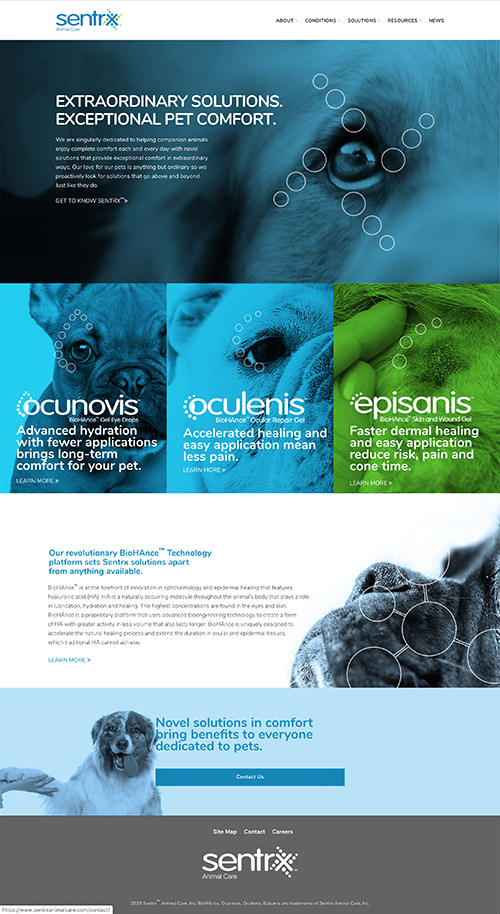The website features a logo in lowercase, with a distinctive blue dot design behind the letter 'X'. The site appears to cater specifically to pet medicine, focusing primarily on dogs. Prominent images of dogs' faces are displayed, and the top navigation bar includes several tabs that are not clearly legible.

The main banner on the homepage emphasizes text that reads, "Extraordinary Solutions, Exceptional Pet Comfort," accompanied by a close-up image of a golden retriever's face, overlayed with the same blue dot pattern seen in the logo.

Below the main banner, there are three highlighted sections, each showcasing images of dogs with colored overlays:

1. **AcuNovus** - "Advanced Hydration with Fewer Applications Brings Long-Term Comfort for Your Pets."
2. **Oculanus** - "Accelerated Healing and Easy Applications Mean Less Pain."
3. **EpiSanus** - "Faster Dermal Healing and Easy Application Reduces Risk, Pain, and Cone Time."

Further down, there is another section with text too small to read clearly, followed by additional graphics.

At the bottom of the page, a message reads, "Naval Solutions in Comfort Bring Benefits to Everyone Dedicated to Pets." The website footer includes links to the site map, contact information, career opportunities, and features a monochromatic version of the Centrix logo along with the text "animal care" against a gray background.